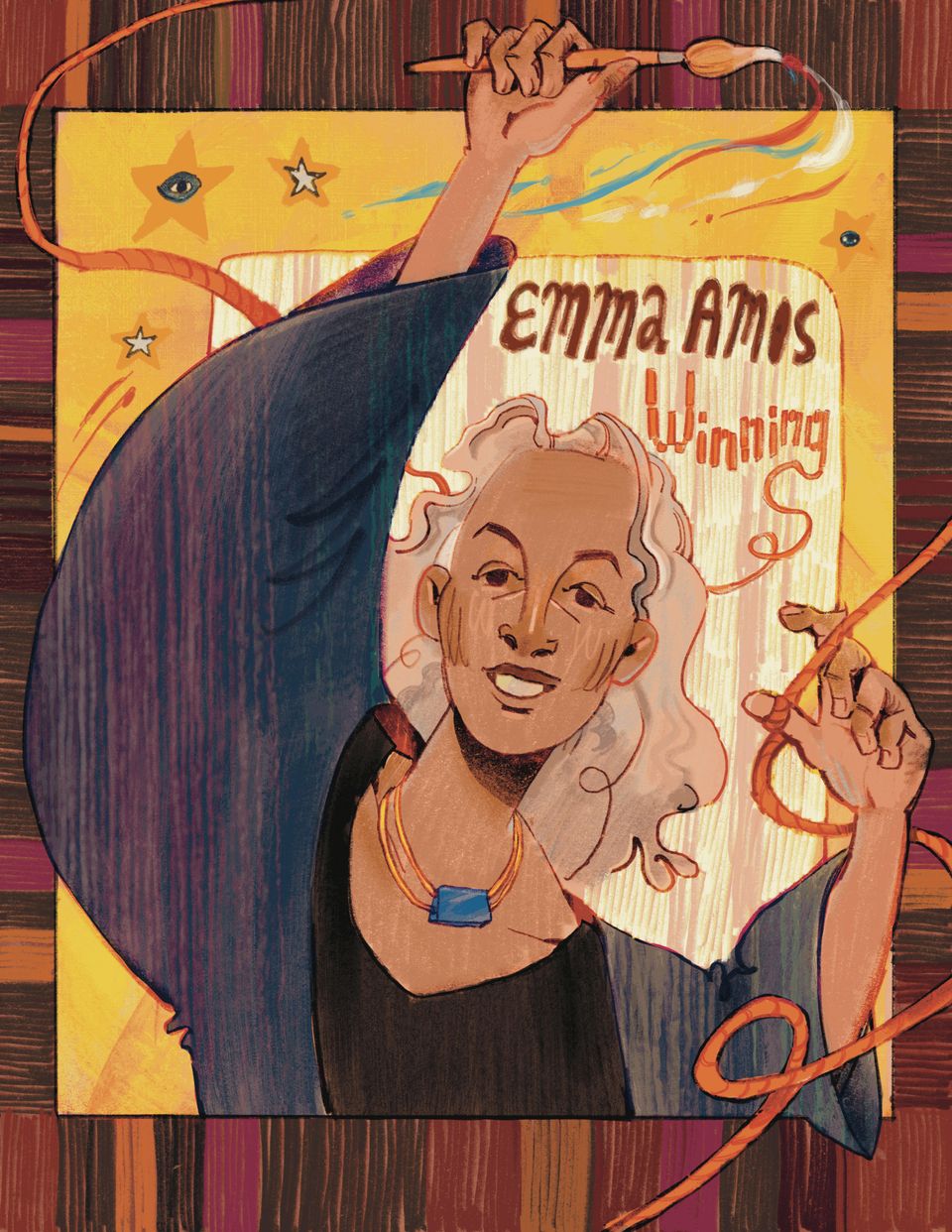The image is a tribute to a joyful woman named Emma Amos, characterized by long, curly white hair. She is smiling and depicted wearing a gold necklace featuring a turquoise gem. Her attire includes a black blouse and a blue-gray fabric, possibly a smock or cape, that drapes over her form and extends up her right arm.

In the scene, she holds a raised paintbrush in her right hand, with colors red, white, and green emanating from it and curving through the yellow rectangular background that frames her. Her left hand is extended, with a piece of twine wound around her thumb and looping around her arm. The twine accentuates the vibrant and dynamic composition, further outlined by a complex background of colors.

The base background is a painted simulation of wooden boards, featuring a palette of browns and reds with varying lines and striations. Yellow and white stars, some small with yellow centers and one larger star containing an eye-like oval, enrich the backdrop. These elements radiate vibrancy and movement, while the words "Emma Amos" and "Winning," written in a rope-like script, are prominently displayed above and below her figure, contributing to the celebratory and artistic essence of the piece.